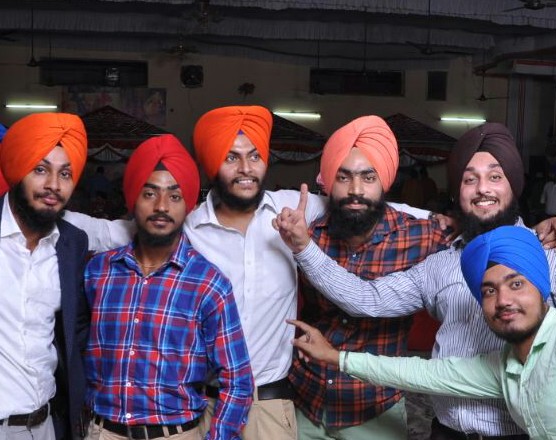In this digital photo taken outdoors, six young East Indian men in their 20s are posing in front of a yellow concrete building with a gray concrete roof. Above them are three evenly spaced, white fluorescent lights and red collapsible roof tents. Each man is wearing a traditional turban: two are orange, one is red, one is salmon pink, one is brown, and one is bright blue. They are dressed in long-sleeve button-up shirts, with one man on the far left wearing a black blazer over a white dress shirt paired with khaki pants. A couple of men in the middle are wearing plaid shirts, one blue and red, another blue and orange. Most of them have thick beards and mustaches, except for one with a thinner beard, and they are all smiling at the camera. Two men on the right are holding up their index fingers in a "number one" gesture. While five men look directly at the camera, the man in the center gazes off to the side. The lively expressions and coordinated attire suggest a celebratory or meaningful occasion, though the exact purpose of the gathering remains unclear.